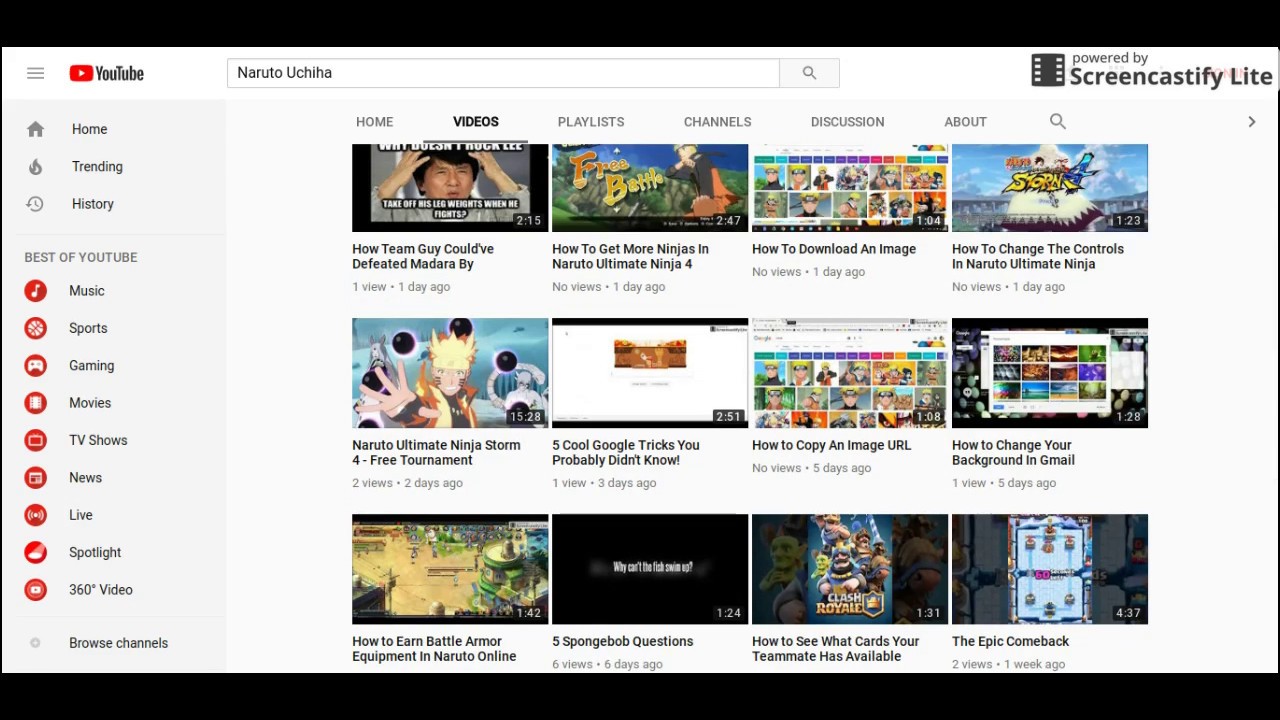In this image, we are observing the YouTube home screen. The top and bottom sections of the image feature a simple black background. In the top left corner, the YouTube logo is displayed prominently, along with a tab menu below it.

Continuing downward, there is a vertical list of categories starting with "Home," followed by "Trending," and "History." Further down, a section labeled "Best of YouTube" is visible with a red icon to the left of each listed category. These categories include "Music," "Sports," "Gaming," "Movies," "TV Shows," "News," "Live," "Spotlight," and "360 Videos." At the very bottom, an option labeled "Browse channels" can be found.

To the right of this vertical list, there are six tabs, with the second one, "Videos," highlighted to indicate the current selection. The tabs read from left to right as: "Home," "Videos," "Playlists," "Channels," "Discussion," and "About."

Below this navigation menu, the main content area displays rows of video thumbnails. There are three rows with four video thumbnails each, totaling twelve videos. The names of these videos are marked in black text, and the video links are positioned at the bottom right corner of each thumbnail.

In the upper right corner of the image, black text reads "Powered by Screen Satisfy Light," accompanied by an emblem resembling a domino, characterized by black with white dots.

Along the left and right edges of the image, two thin vertical black lines frame the entire screen, creating a defined outer barrier.